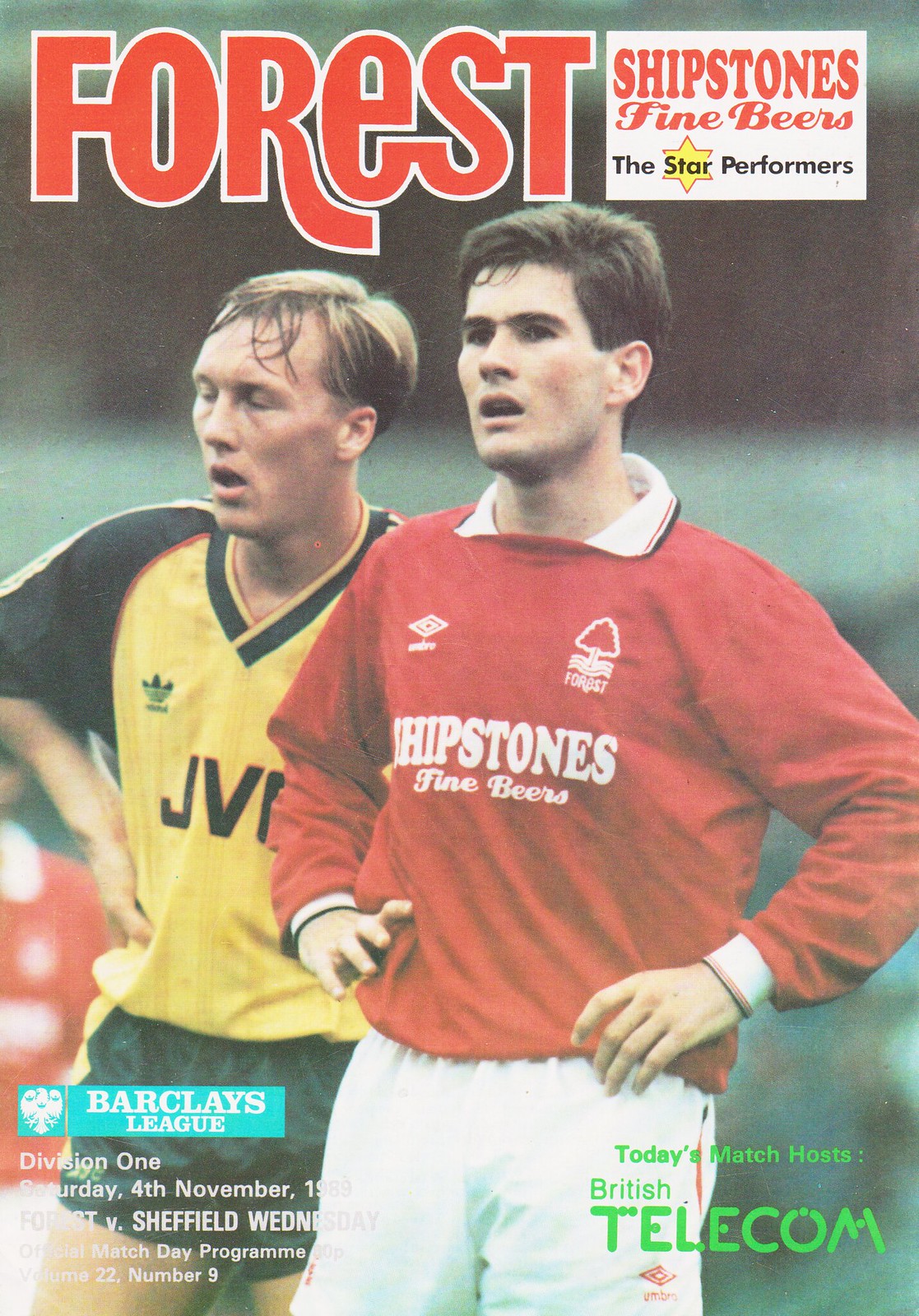This detailed image features the cover of an official match day program from the Barclays League Division 1, dated Saturday, November 4th, 1989, highlighting a soccer game between Nottingham Forest and Sheffield Wednesday. The central focus is on two soccer players: the player representing Nottingham Forest is centered, wearing a red jersey with white shorts, and has "Ship Stones Fine Beers" emblazoned on his jersey. He is a white male with black hair, standing with hands on his hips. Behind him, to the right, is a Sheffield Wednesday player dressed in a yellow and black jersey with "JVC" displayed on it. 

The background includes several textual elements and logos: in the top right corner, "The Star Performers" is prominently featured with a star graphic. The bottom left corner houses the Barclays logo. Further textual information includes "Forest, Ship Stones, Fine Beers, The Star Performers, Barclays League, Division 1, Saturday 4th, November 1989, Forest vs. Sheffield Wednesday, Official Match Day Program, Volume 22, Number 9." Additionally, "Today's Match Host British Telecom" is noted on the right-hand side. Color highlights include red and white for Forest’s jerseys, black and yellow for Sheffield’s jerseys, green text for British Telecom, and light blue elements associated with the Barclays branding, capturing the essence of a quintessential English soccer match program from the late 1980s.